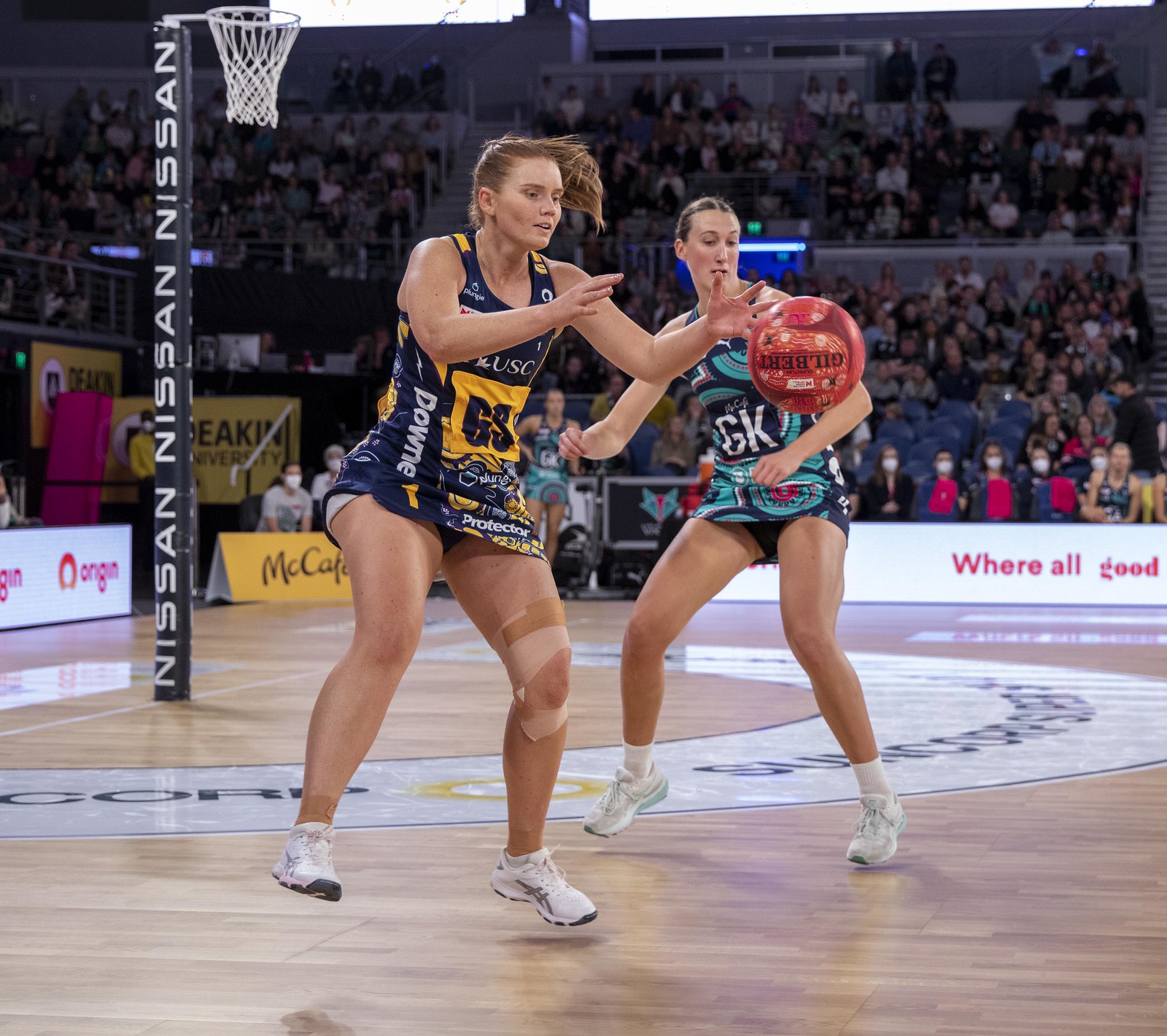This detailed image captures a women's netball game on a hardwood court with a crowd of masked spectators in the background. The player on the left is depicted mid-air with her long, straight brown hair flowing to the side, as she reaches out to catch a red and pink ball. She is wearing a sleeveless navy blue dress with yellow accents and the number 63 prominently displayed in the center against a yellow square. To her right, another player dressed in a blue and green outfit with 'GK' in white lettering against a dark blue square is also slightly off the ground, indicative of the dynamic movement in the game. The scene is set under a basketball goal with "Nissan" written above it multiple times. The court features light brown brick tiles, enhancing the competitive atmosphere.